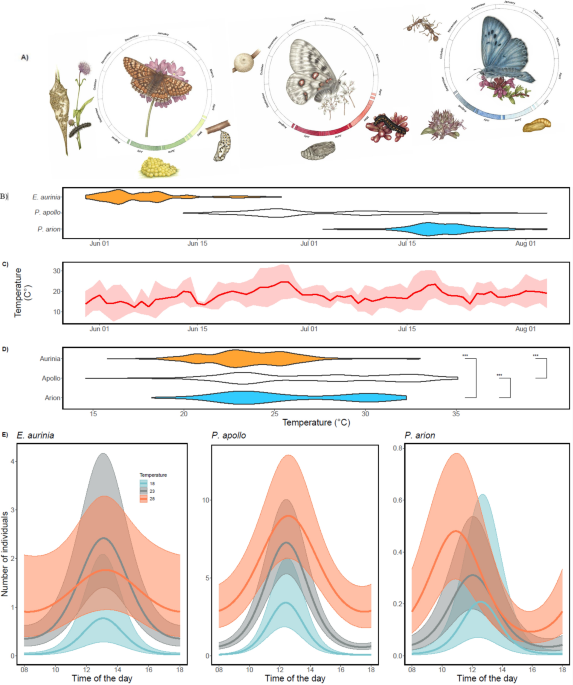This image is a detailed, colorful diagram from a scientific paper on butterflies and moths, illustrating their characteristics and activity patterns. At the top, labeled "A", it features three distinct butterflies: an orange and black striped moth on the left, a white moth with black stripes and red dots in the center, and a blue butterfly with black dots on the right, each placed alongside flowers and green stems. There are also various items beneath these insects, such as cocoons, larvae, and ants.

Below the main illustrations, the diagram is divided into several sections labeled "B", "C", and "D". Section "B" contains a time-bound representation of the lifespans of the insects, shown as orange, white, and blue blobs. 

Section "C" features a red line graph that represents temperature fluctuation, surrounded by a pink outer edge indicating the temperature range.

Section "D" has another spread of orange, white, and blue blobs, similar to section "B", possibly depicting different stages in their life cycles or movements.

The bottommost section includes four rectangular line graphs, each depicting the number of individuals active at different times of day. These graphs are color-coordinated in blue, orange, white, and red, and underscored by the themes of time and frequency of activity. The background of these graphs is white, providing a contrast to the vibrant pastel colors throughout the rest of the diagram which includes peach, blue, tan, and darker blue tones. This beautifully illustrated representation is rich with specific details about different butterfly species and their behaviors, outlined meticulously for scientific analysis.